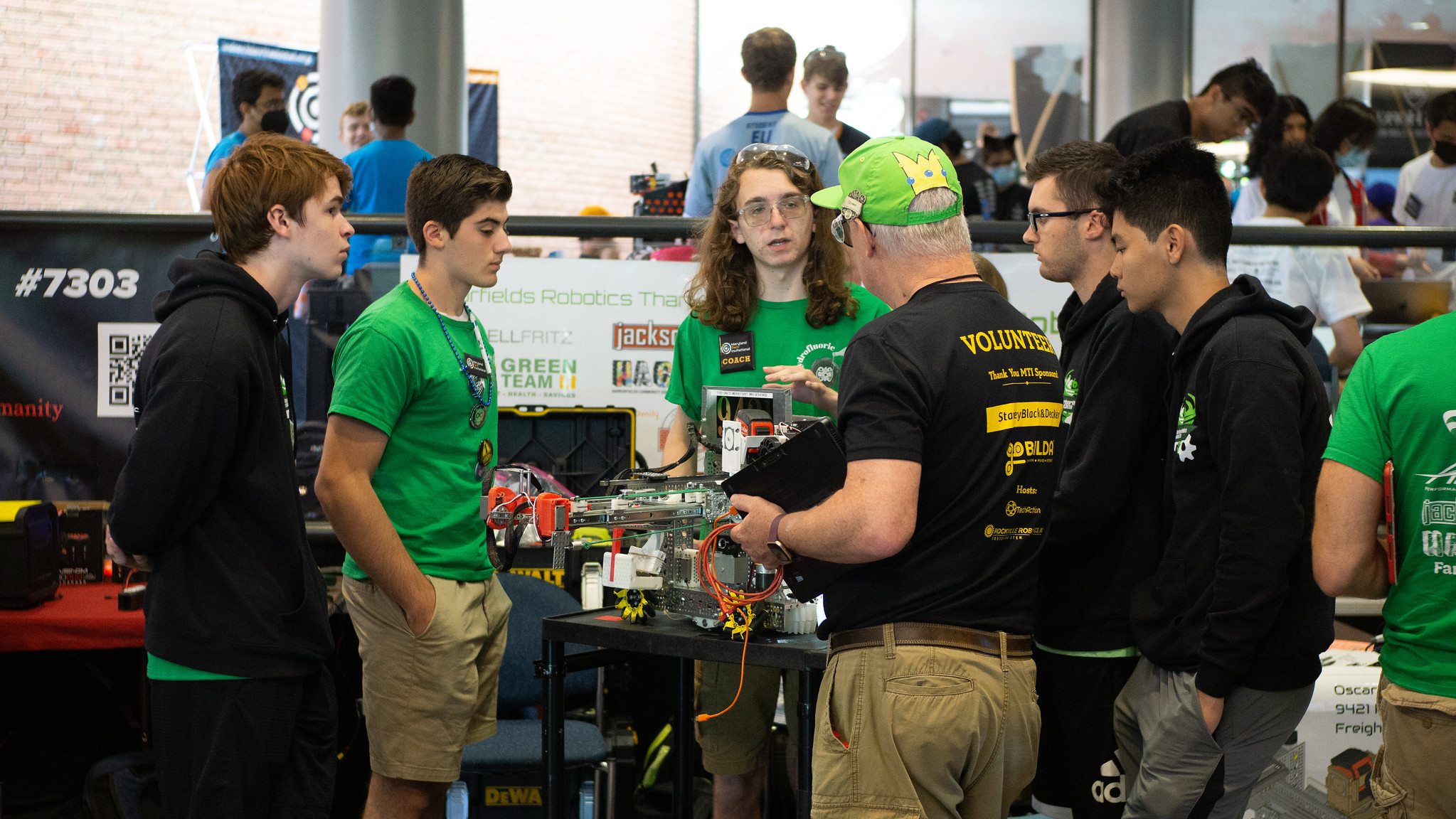In this image, a group of six teenagers, composed of boys and one girl, are gathered around an older man who appears to be in his fifties or sixties. The man, dressed in a bright green baseball cap and a black shirt with yellow writing on the back that reads "volunteer," is explaining how an electrical device works. He also holds a bundle of wires and a laptop, suggesting a hands-on demonstration. The teenagers, wearing green t-shirts and some in black hoodies with green designs, are listening attentively. The setting seems to be a science competition or educational fair, as indicated by the banner in the background displaying various company names, and other teams wearing different colored shirts. A window is visible in the background, adding to the indoor environment. Some of the boys have their hands in their pockets, and there are other children scattered in the background, creating a busy and engaged atmosphere.